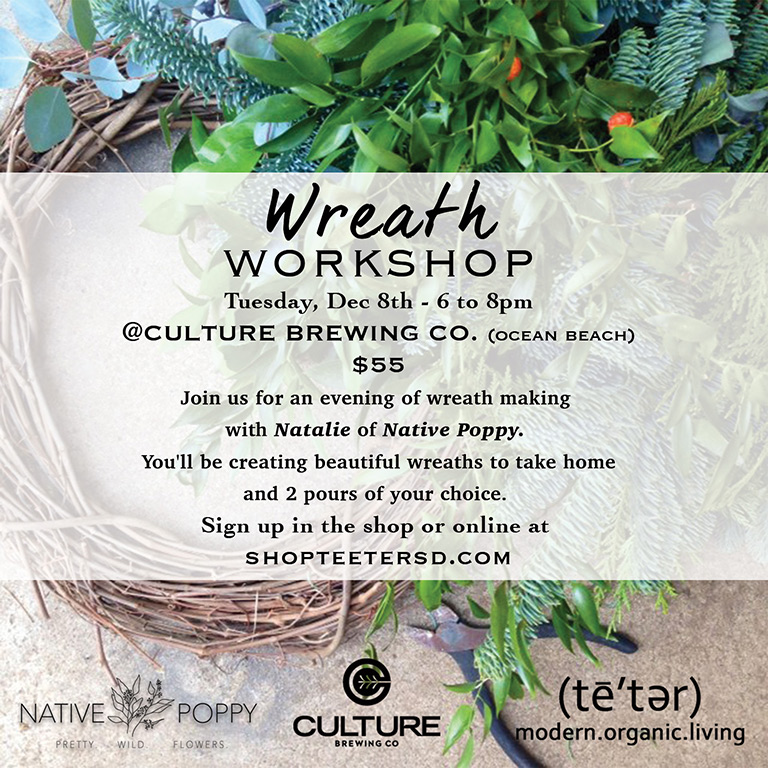The poster is an advertisement for a wreath workshop featuring a detailed and inviting background of various wreath-making items. Toward the left and center of the image, there's an undecorated grapevine wreath made of twisted twigs. Eucalyptus sprigs and lush green pine branches are visible toward the upper center, symbolizing the natural elements you'll use in the workshop. A transparent, light tan banner with black text overlays the center of the image, announcing the event: "Wreath Workshop, Tuesday, December 8th, 6 to 8 p.m. Culture Brewing Company, Ocean Beach, $55." The text invites you to join Natalie of Native Poppy for an evening of crafting beautiful wreaths to take home, complemented with two pours of your choice. Details about signing up are provided, directing you to the shop or online at shopteetersd.com. At the bottom of the image, spanning from left to right, logos of three sponsors, including Culture Brewing Company and Native Poppy, are displayed, adding credibility and partnership to the event. Additionally, a metal plant clipper is subtly placed in the background, enhancing the theme of creative tools at your disposal.